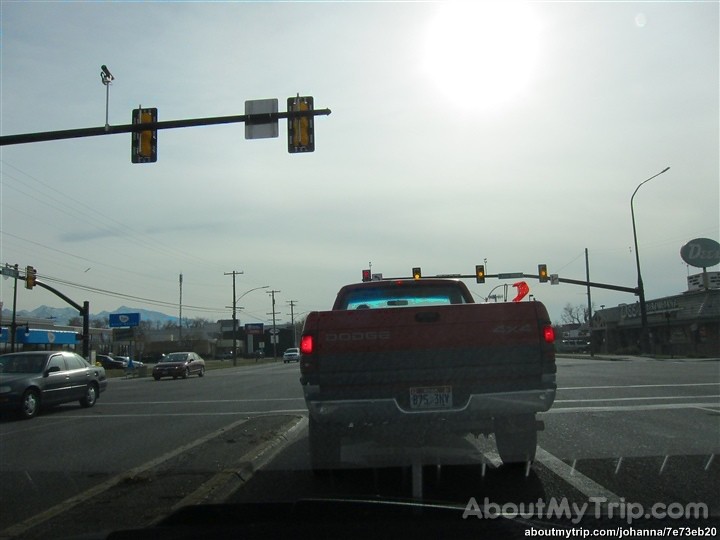The image is dash cam footage taken from inside a car, depicting an outdoor scene at a large T-junction intersection. The windshield frames a red Dodge 4x4 pickup truck in the lane ahead, with its chrome bumper and gray trim visible. The truck's brake lights are on, and above it, a traffic light shows a red signal. In the other three lanes beside the truck, traffic lights are displaying yellow signals. On the left, several cars, including a sedan of indeterminate color, are passing by the stationary truck. The background features various establishments; to the right is a restaurant with a sign that reads "Dee's," and to the left, an intersection with a store that appears to be a Napa Tires. The scene includes multiple street lamps and traffic lights, capturing reflections off the car's windshield, and the sky, which is mostly clear with some clouds. At the bottom right of the image, the watermark "aboutmytrip.com" and a link "aboutmytrip.com/johanna" are visible, the latter possibly including an identification code or number.